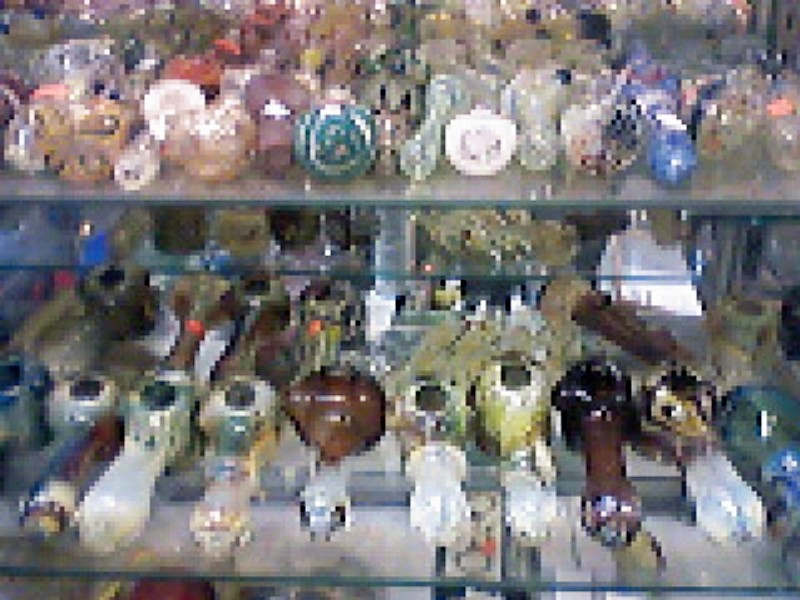This highly pixelated and blurred photograph, possibly a video screen capture, depicts a glass pipe display within a store setting. The display features two visible clear glass shelves, each laden with an array of blown glass items ranging in color from browns and blues to clear, with some hints of vibrant tail colors and light oranges. Despite the poor image quality, some pieces appear to have distinctive shapes characteristic of bongs or possibly perfume bottles, featuring elongated necks leading into circular bases. Bright orange price tag stickers are faintly visible, providing a clue to the retail environment. Although the image is too grainy to discern specific details, the variety of colorful, decorative glass items and their positioning in clear, glass shelving showcase an intricate and likely vibrant assortment of either smoking apparatus or perfume containers.